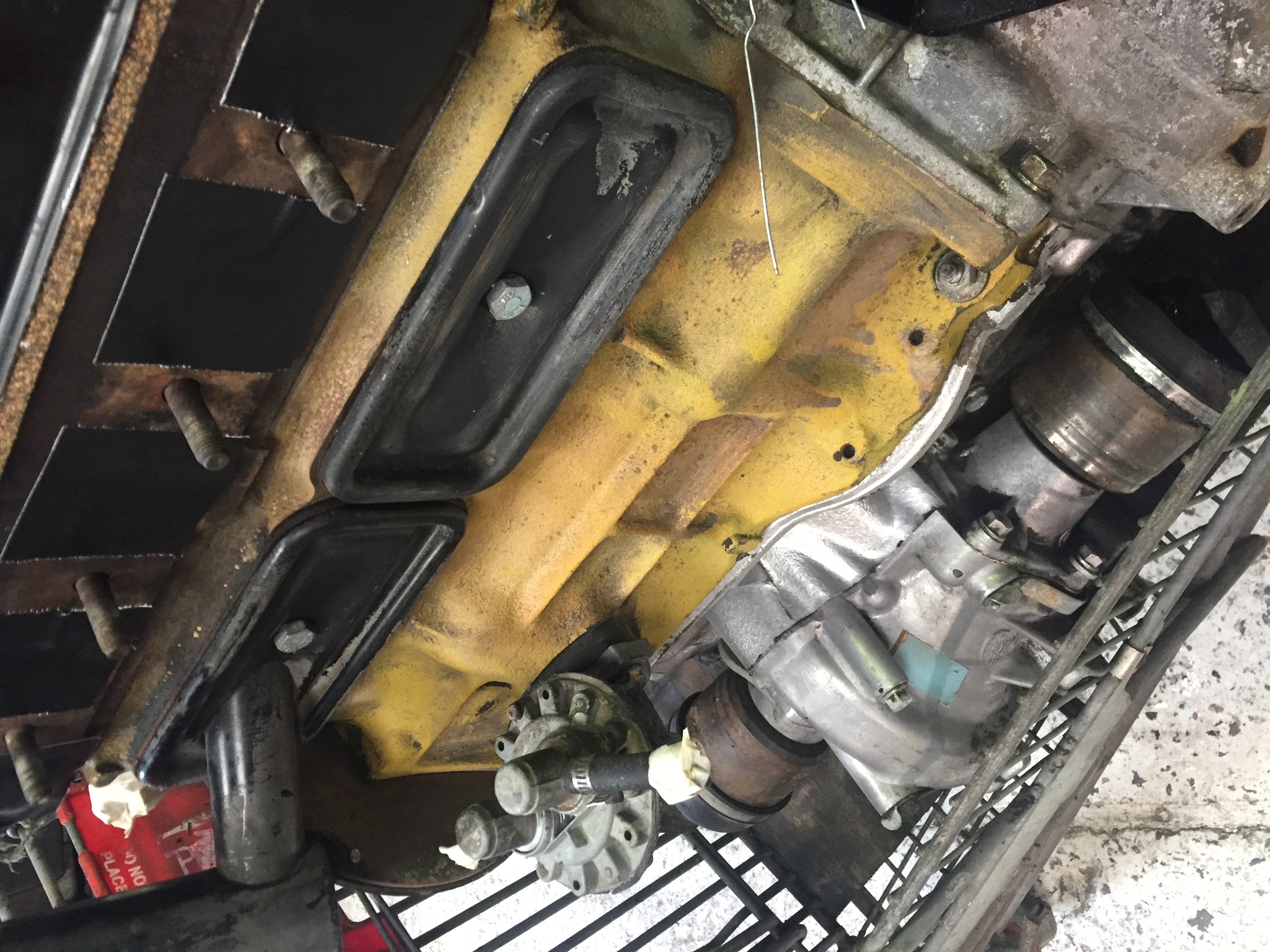The photograph intricately captures the underside of a mechanical structure, which might be part of a vehicle or possibly a metal cart used for holding various tools and metal pieces. On the far left of the image, there is a gray metal bar, followed by a long brown piece adjacent to it. Next to the brown piece, there is a darker metal component, featuring several screws or bolts protruding from it. Running parallel to this darker metal piece is another metal bar, transitioning in color from a darker shade at the bottom to a dirtied yellow towards the top.

Centrally positioned within the image is a gray, almost black, metal plate with a screw or bolt fixed in its center. Below it lies a similar metal plate. To the right of these plates is a larger yellow metal component, distinguished by screws or bolts at its top left and top right corners. Beneath this large yellow piece is a gear-like element. At the upper part of the image, above the gear, there is a larger metal assembly featuring various colors and housing two small wheels on either side, with a lighter gray segment in its middle. The overall composition of the image offers a detailed glimpse into a complex mechanical assembly with a variety of metal components and fastenings.